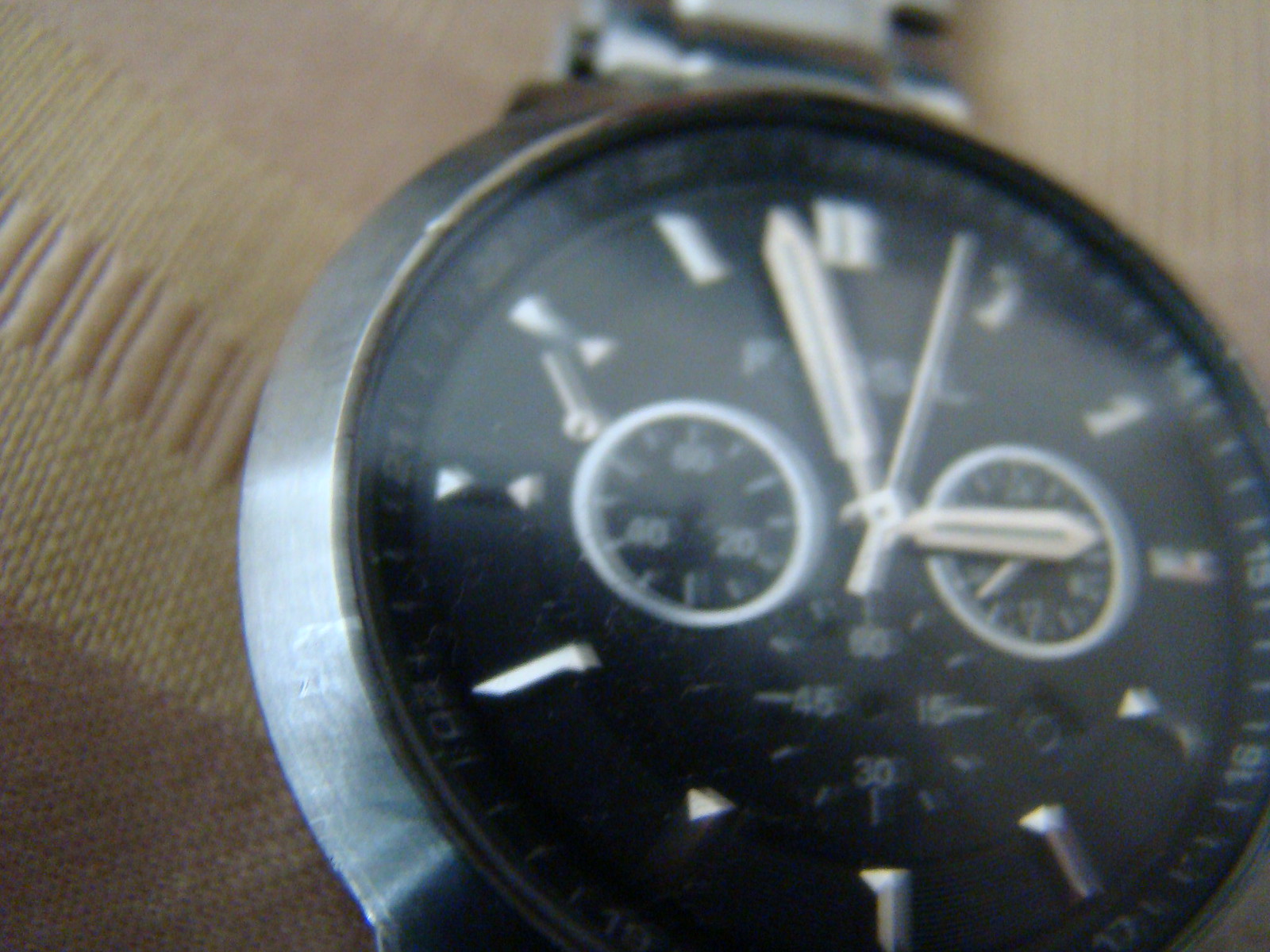A detailed close-up image showcasing a wristwatch placed on top of a fabric with brown and tan stripes. The watch features a silver stainless steel frame and a matching stainless steel wristband, both exuding a sleek and modern appearance. The face of the watch is striking with its black background, adorned with two prominent white circles centrally positioned. At the bottom of the face, there is a gauge marked with white numerical indicators. Surrounding the face are silver or white numerical markers, enhancing the timepiece's readability. The watch also has two sturdy, silver-colored hands and a thin, more delicate third hand positioned at the center, contributing to its precise time-telling functionality. The overall composition of the watch against the striped fabric creates an appealing contrast, highlighting the craftsmanship of the timepiece.